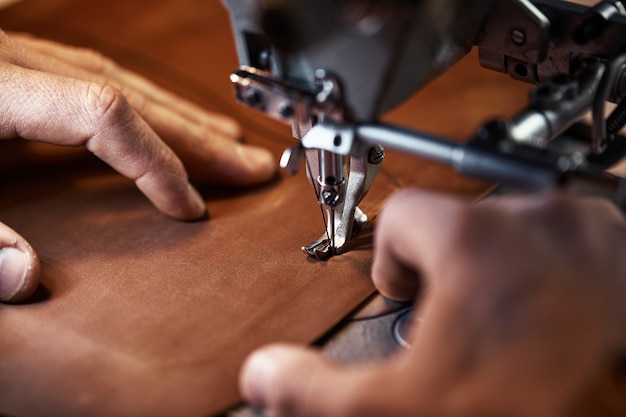The image depicts a close-up view of a person with light skin using a sewing machine. Both their left and right hands are holding and guiding a piece of medium brown, textured fabric—possibly cotton—through the machine. The right hand appears slightly blurry and is positioned near the right edge of the image. In the upper right corner, extending down towards the center, is the arm of a silver sewing machine, with a visible needle threaded with black sewing thread. While the sewing machine itself appears a bit blurry, you can still discern the machinery and additional details in the background. The overall image is in color, well-lit, and clear, highlighting the intricate process of sewing.